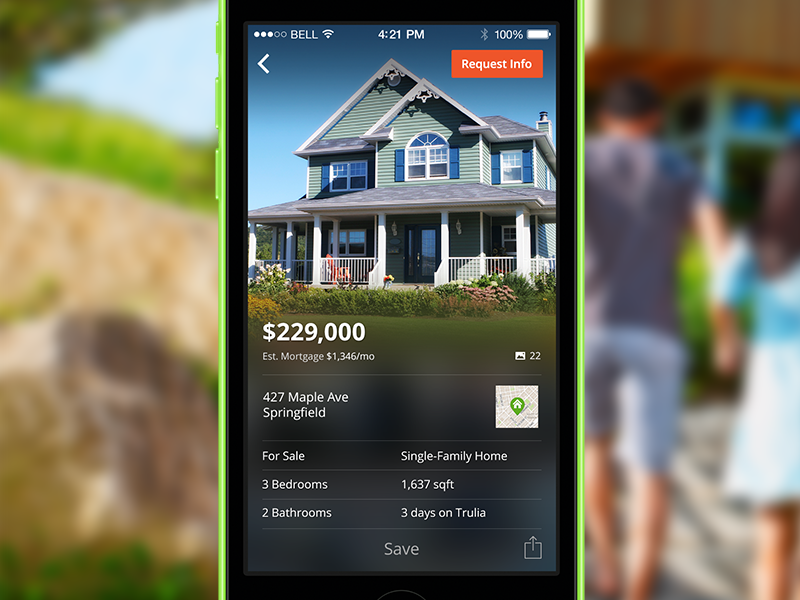The advertisement prominently features a bright green smartphone displaying a real estate listing. The phone screen shows the time as 4:21 PM and indicates a full battery at 100%. In the top right corner, an orange rectangle with the text "Request Info" in white stands out. Below this, there is a photo showcasing the front of a house with a price tag of $229,000. The estimated mortgage for the property is listed as $1,346 per month. A small note indicates that there are 22 photos available for viewing.

The address of the property is 427 Maple Avenue, Springfield. The house is described as a single-family home for sale, featuring three bedrooms and two bathrooms, with a total living area of 1,637 square feet. The listing has been posted on Trulia for three days. At the bottom center of the phone screen, a gray "Save" button is visible.

In the background of the image, there is a blurred-out scene. On the right side, two people appear to be walking up a set of stairs, while on the left side, a grassy hill is faintly visible, adding context to the setting of the advertisement.